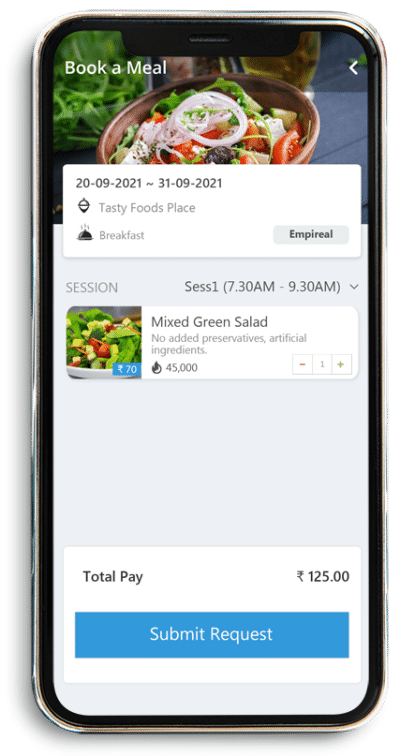Displayed is an image portraying a mobile phone’s screen featuring a food delivery or booking app. The screen’s header displays the title "Book a Meal," accompanied by an appetizing image of a bowl filled with salad greens resting on a gray table, accented by additional greens and dressing in the background. Directly beneath this section, a date range is visible: "2009-2021 through 3109-2021" from "Tasty Foods Place," specifying the breakfast service category labeled "Imperial."

Further down, the app details the available session, "Session 1," occurring from "7:30 AM to 9:30 AM." Below this session information is another visually appealing image of a mixed green salad. The description mentions the absence of added preservatives and artificial ingredients, alongside an extraordinary price tag of "$45,000." The quantity indicated as selected is "1."

At the bottom of the screen, the app displays the total payment amounting to "125" and provides a button to "Submit Request."